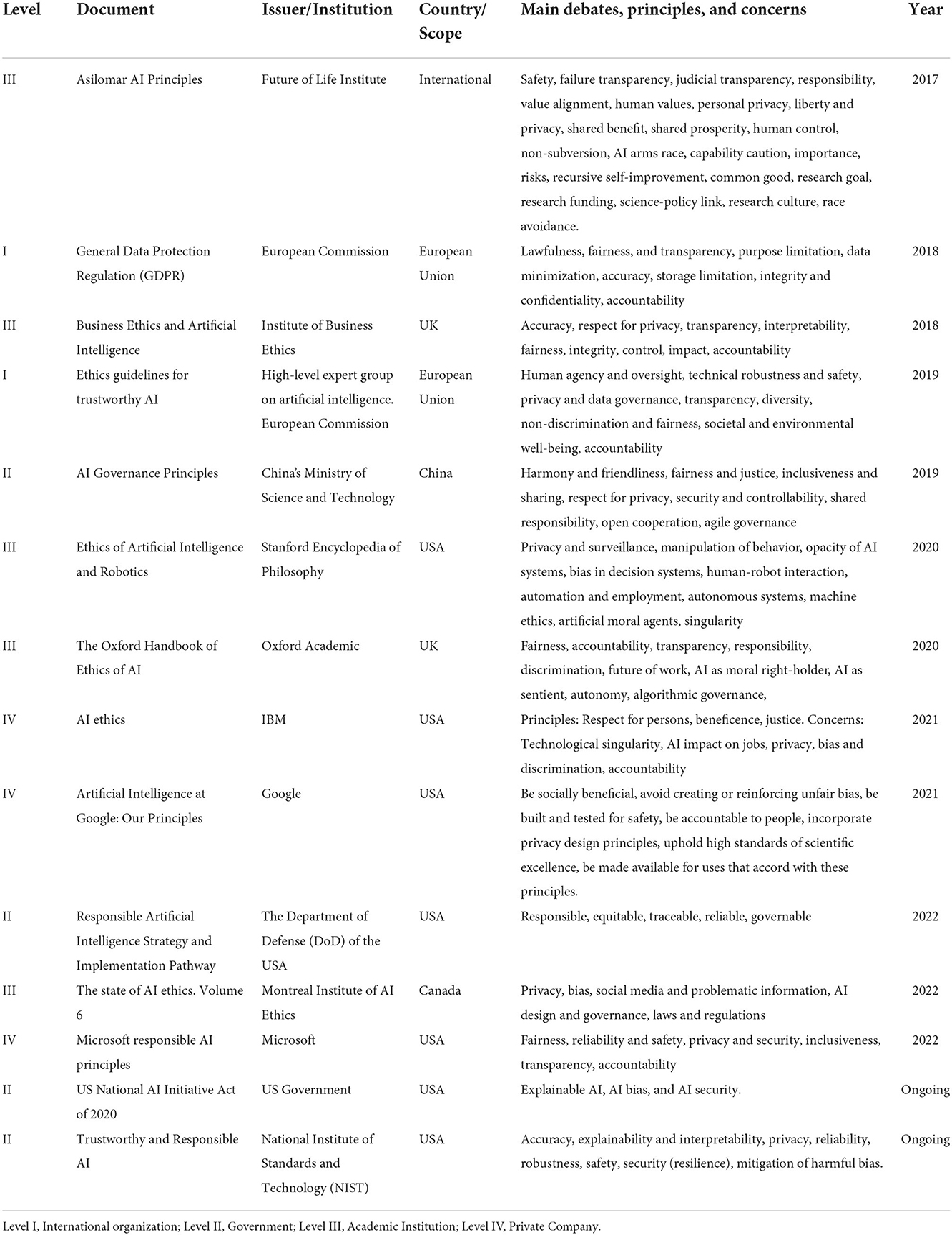The background of the image is white. Along the top part of the image, there is a bold heading that reads: "Level, Document Issuer/Institution, Country/Scope, Main Debates, Principles, and Concerns, Year." Below this heading is a thin gray line separating it from the content beneath.

Below the gray line, the content is divided into multiple columns containing data that looks like Roman numerals and other information. Specifically, the levels are arranged as follows: III, I, III, I, II, III, III, IV, IV, II, III, IV, II, II. 

The documents listed are:
1. ISOMAR AI Principles
2. General Data Protection
3. Business Ethics and Artificial Intelligence
4. Ethics Guidelines for Trustworthy AI
5. AI Government Principles
6. Ethics of Artificial Intelligence and Robotics
7. The Oxford Handbook of Ethics and AI
8. Ethics of Artificial Intelligence at Google
9. DoD Principles
10. Responsible Artificial Intelligence Strategy
11. Implementation Pathway
12. The State of AI Ethics, Volume Six
13. Microsoft Responsible AI Principles
14. US National AI Initiative Act of 2020
15. Trustworthy and Responsible AI

Each document is attributed to different issuers or institutions:
1. Future of Life Institute
2. European Commission
3. Institute of Business Ethics
4. High-level Expert Group on Artificial Intelligence (European Commission)
5. China's Ministry of Science and Technology
6. Stanford Encyclopedia of Philosophy
7. Oxford Academic
8. IBM
9. Google
10. DoD (Department of Defense, USA)
11. Montreal Institute of AI Ethics
12. Microsoft
13. US Government
14. NIST (National Institute of Standards and Technology, USA)

The country or scope indicated for each document is as follows:
1. International
2. European Union
3. UK
4. European Union
5. China
6. USA
7. UK
8. USA
9. USA
10. USA
11. Canada
12. USA
13. USA
14. USA

The years of publication are:
1. 2017
2. 2018
3. 2018
4. 2019
5. 2019
6. 2020
7. 2020
8. 2021
9. 2021
10. 2022
11. 2022
12. 2022
13. Ongoing
14. Ongoing

Overall, the image seems to present a structured and detailed overview of various AI ethics-related documents, their issuing bodies, geographical scope, and publication years, organized in a table format.